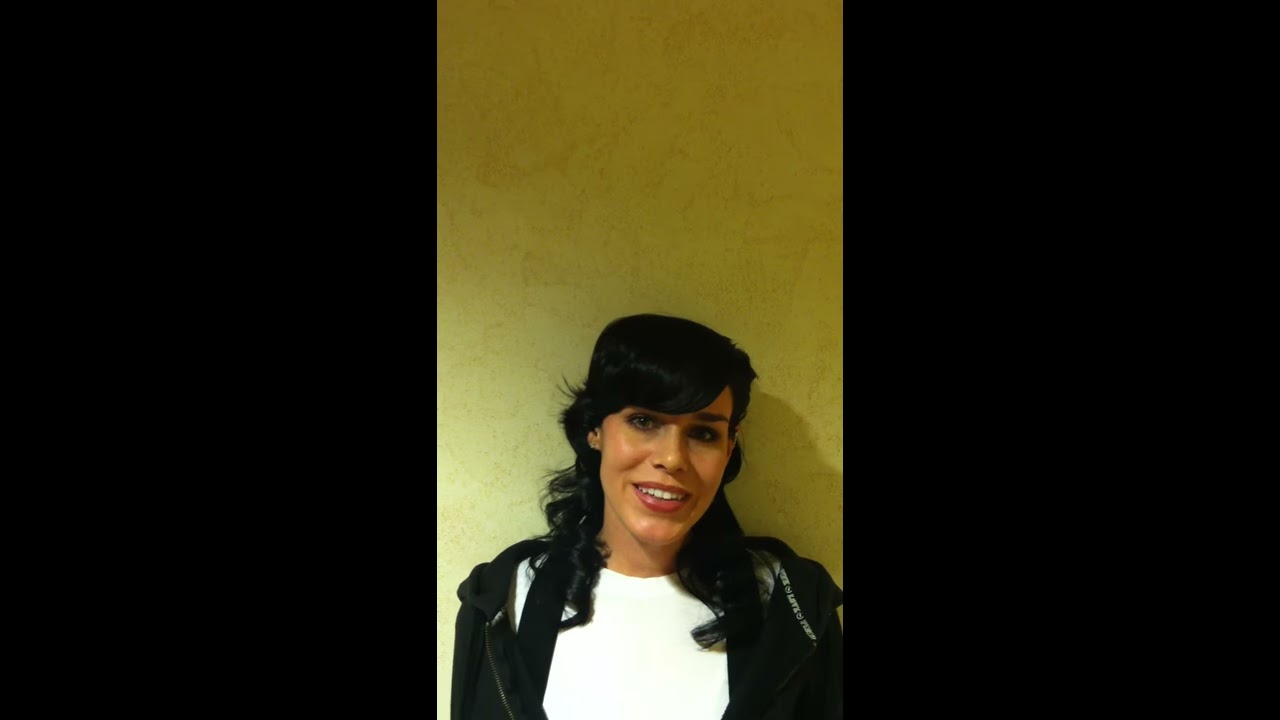In this image, we see a young woman, likely in her 20s or 30s, smiling warmly with her top teeth visible. She has dark, curly black hair with bangs that fringe her forehead and falls around her shoulders. Her eyes are dark brown, and she wears earrings. Her complexion is a tan shade. She is dressed in a white shirt layered with a black hooded jacket that bears white lettering on the lining at the neckline, though the text is unclear. There are black straps that resemble overall straps crossing over her white shirt. 

The backdrop is a beige or yellow wall with some random marks and smudges, indicating a lived-in space, possibly an interior setting like a home, office, or school. She is seated against the wall, and there is a noticeable shadow cast behind her, adding depth to the image. The primary colors in the photograph are yellow, white, and black, contributing to a visually striking yet simple composition.